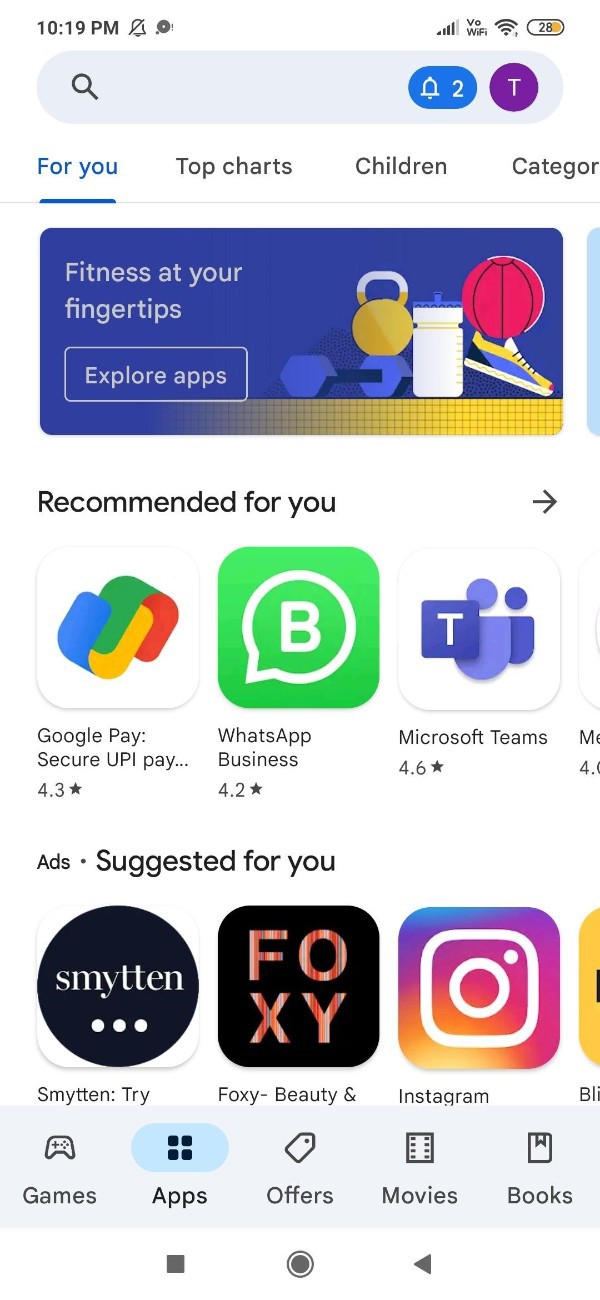The image is a screenshot taken from a mobile phone device, capturing a view of an application store, akin to the Google Play Store. At the top of the screen, various status icons are visible, including the time, network connection, WiFi signal, and battery life. Below these indicators, a grey, empty search bar is prominently displayed.

The top section of the screenshot features navigation options labeled "4U," "Top Charts," "Children," and "Categories," with the "4U" section being highlighted. Dominating this section is a rectangular graphic showcasing smaller images of exercise-related equipment such as trainers, a water bottle, a kettlebell, a dumbbell, and a basketball, accompanied by the text "Fitness at your fingertips." Beneath this graphic is a rectangular button with the text "Explore apps."

Further down, the "Recommended for you" section displays various application thumbnails. Each thumbnail includes the app icon, the application name, and its rating.

At the bottom of the screenshot, additional navigation icons segment the app store into various categories, including "Games," "Offers," "Movies," and "Books."